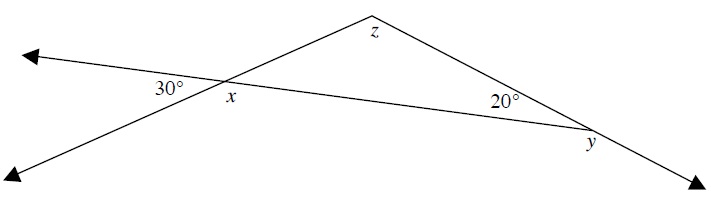The image features a complex arrangement of intersecting lines with arrows at their tips, forming multiple triangles. The central focus is an irregular, non-equilateral triangle prominently displayed in the center. Within this triangle, the internal angle at the right vertex is explicitly marked as 20 degrees. To the left side of the image, additional lines intersect to form the two visible sides of another triangle, although its third side extends beyond the frame. This triangle has an internal angle labeled 30 degrees at its visible vertex.

Extending from these intersections, arrows indicate the direction of the lines: one arrow points leftward, two others point downward and to the lower left, while another points downward and to the right from an apex, suggesting a dynamic flow of directions. Each corner of the central triangle is annotated with a letter: 'Z' at the top vertex, 'X' at the left vertex, and 'Y' at the right vertex. The entire composition is set against a white background, emphasizing the clarity and precision of the geometric lines and annotations.